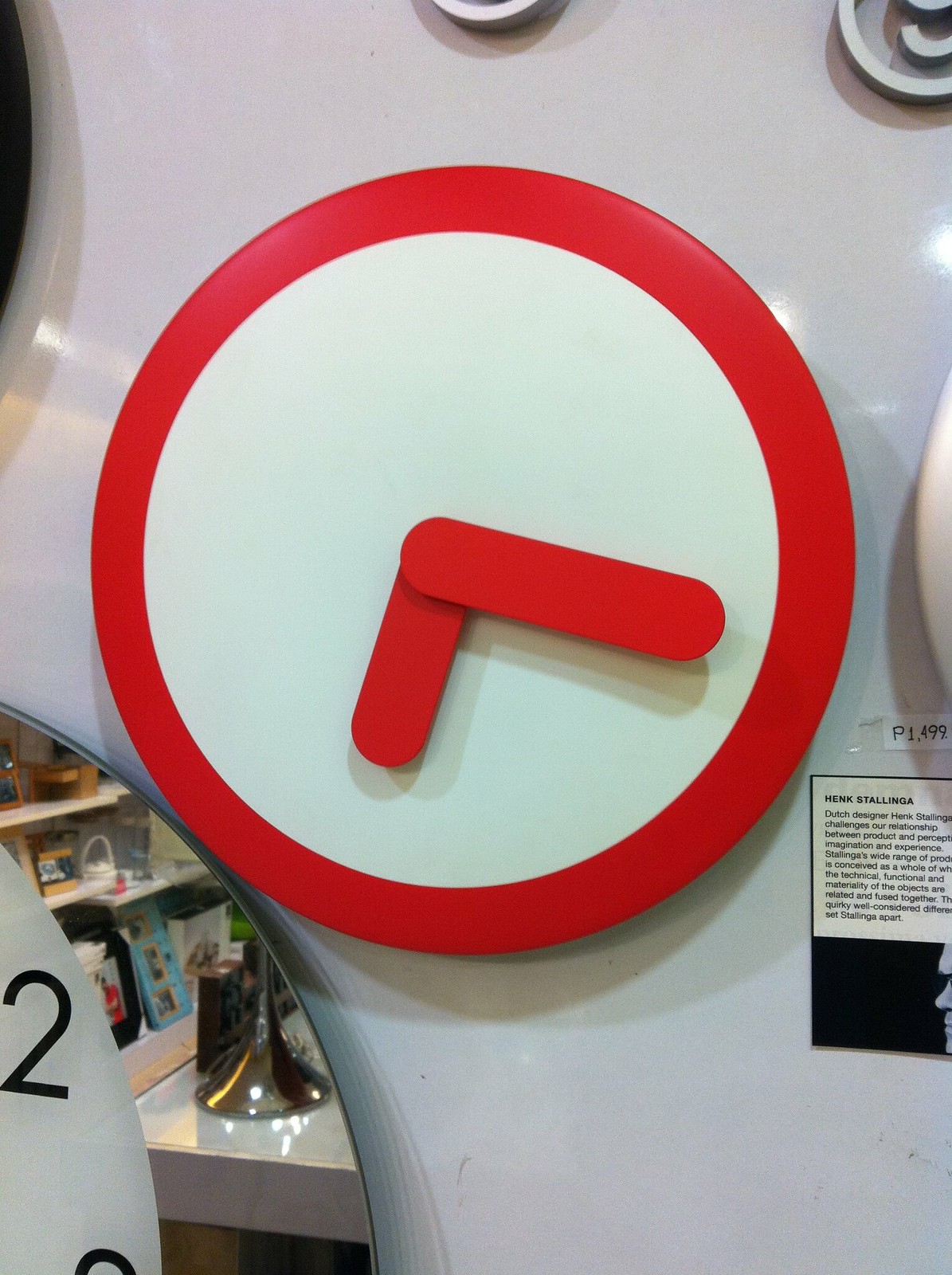The photograph captures a sleek, indoor display of various clocks mounted on a high-polished, white metal surface. Central to the image is a modern, round, analog clock characterized by its minimalist design—devoid of numbers. The clock's face is a stark, clean white, while its exterior rim and both the minute and hour hands are a vivid, matching red. Adjacent clocks, one partially visible with a mirrored rim, add depth and complexity to the visual arrangement, creating an intriguing and sophisticated clock showcase.